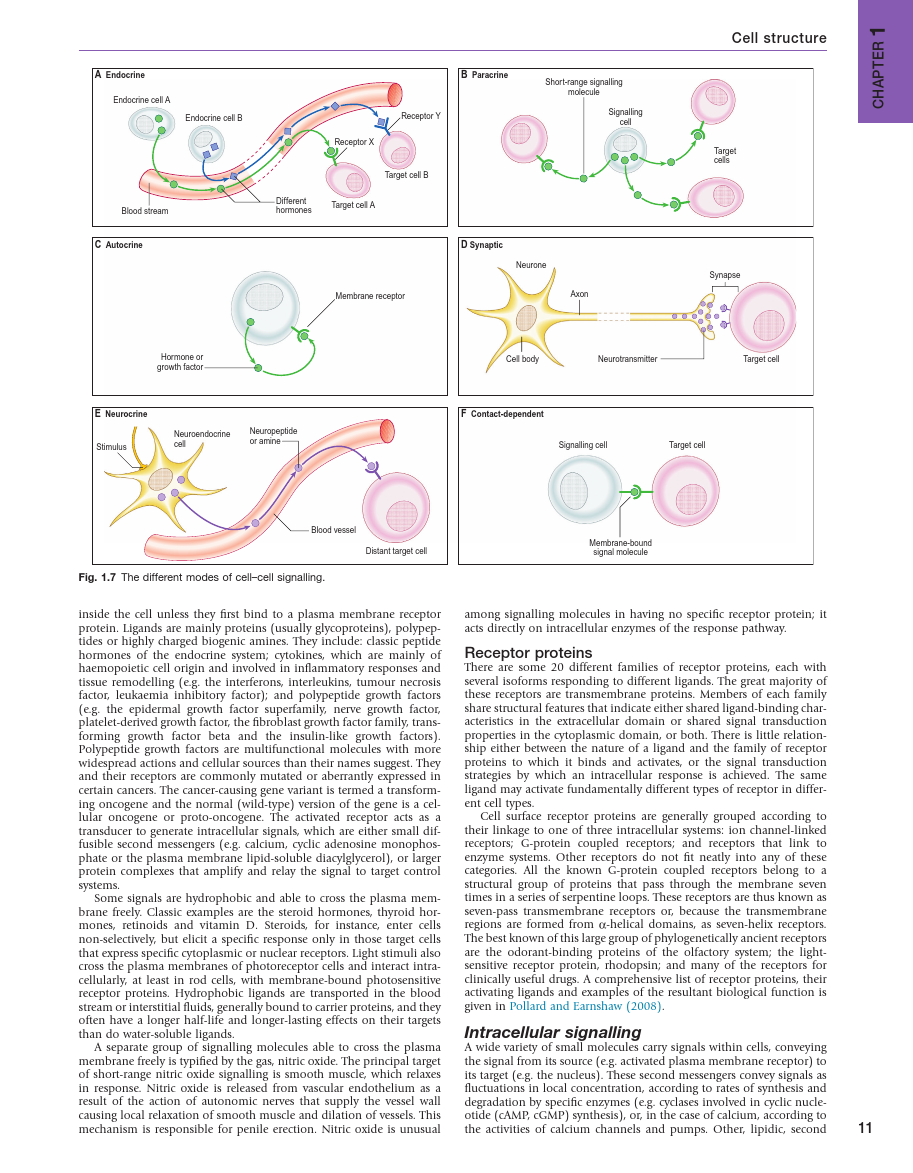This photograph captures a page from an educational biology textbook, specifically from Chapter 1 titled "Cell Structure." In the top right corner, "Chapter 1: Cell Structure" is subtly noted in small print. The main focus of the page is a comprehensive illustration labeled "Figure 1.7: The Different Modes of Cell Signaling." The drawings are rendered in various colors, including orange, light orange, pink, green, and yellow, set against a white background. Below these detailed illustrations, explanatory text elaborates on the figure. 

The page features six distinct illustrations of cell signaling mechanisms. On the top left, there’s an illustration of endocrine cells (labeled as Endocrine Cell A and Endocrine Cell B), depicted as round cells with arrows indicating hormone movement through the bloodstream, highlighting their interaction through veins or arteries. To their right, paracrine cells are also represented as round structures demonstrating their signaling molecules' roles. The synaptic cell, illustrated next, is a spiky model showing nerve cells sending signals to target cells. Autocrine cells appear to create hormones, while neurocrine cells are shown sending signals to the blood. Lastly, the contact-dependent signaling model highlights interactions through direct cell contact. The accompanying text panel provides an in-depth explanation of each cell type and their respective signaling functions, suggesting that this page is intended for a college-level audience.